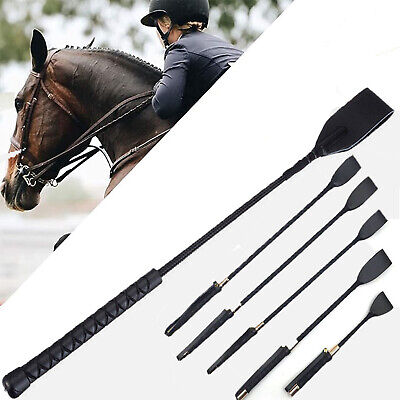The image is an advertisement showcasing six different riding crops of varying styles and lengths, arranged in descending order from largest to smallest. Each crop features a rubber handle and a leather or rubber tip, indicating their specialized usage for increasing speed during racing or jumping. On the left side of the image, there is a jockey dressed in English riding attire, including a helmet and a shirt, riding a dark-colored horse with a short mane and full riding gear. The jockey appears to be in complete control of the horse, whose head and upper body are visible. The image is divided in a way that emphasizes both the detailed features of the jockey and horse as well as the intricacies of the riding crops, appealing to those interested in equestrian equipment.